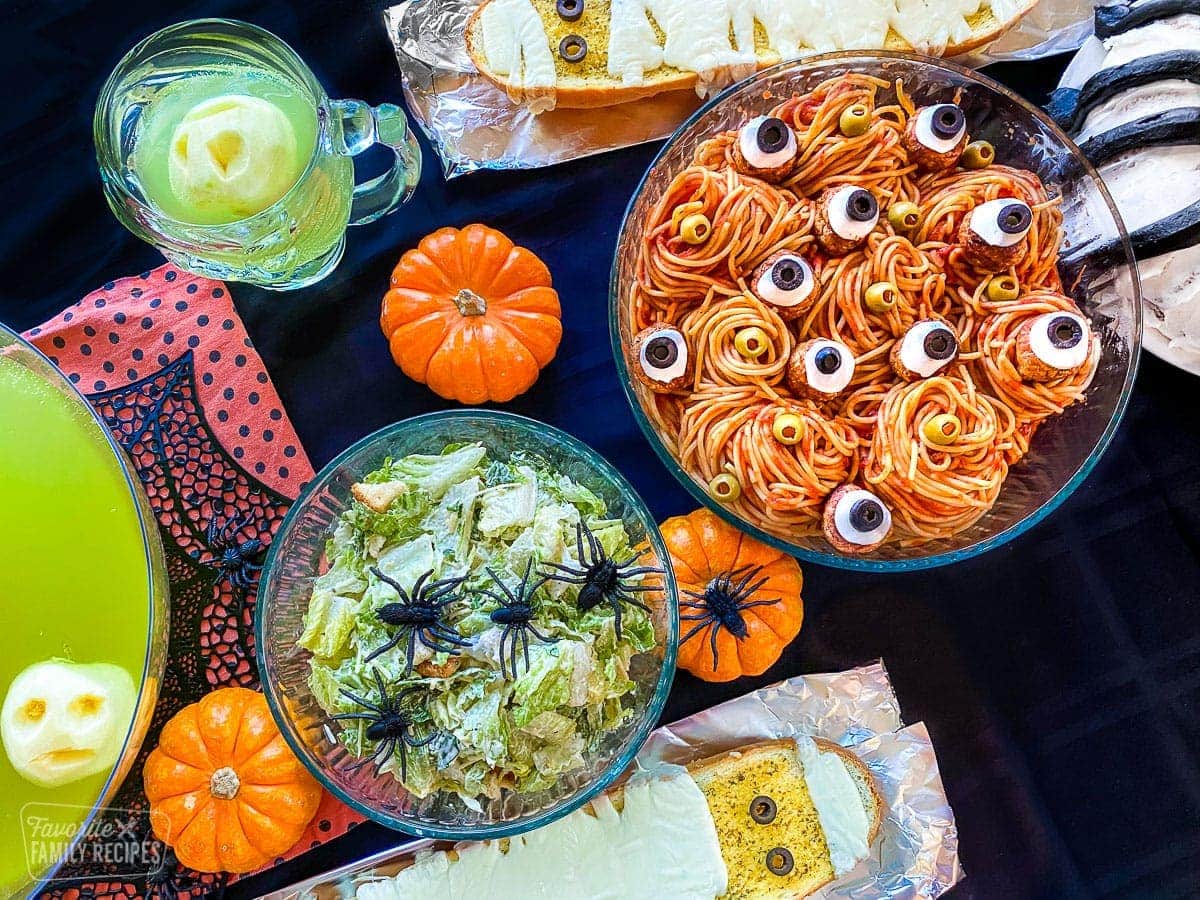This is an aerial view of a Halloween-themed food display set on a black tablecloth. The spread includes various spooky dishes intricately arranged for a festive atmosphere. Prominent elements include small pumpkins, one of which features a spider atop it, enhancing the eerie decor. There is a Caesar salad sprinkled with four black fake spiders, adding to the spooky feel. A bowl of spaghetti is garnished with eyeball-like creations made from ricotta cheese and olives, with additional loose green olives mimicking eyeballs scattered around. Green punch in a punch bowl appears almost as if it's glowing, casting an otherworldly vibe. A mug of the same concoction features ghost-patterned ice cream, designed with eyes and a face to embody a spectral presence. Pieces of garlic bread decorated to resemble mummies, complete with olive eyes and heavy cheese patterns, are positioned both at the top and bottom of the image. The setting also includes detailed stainless steel cutlery with black, Halloween-themed bases, tying the display together into a cohesive, spooky feast.